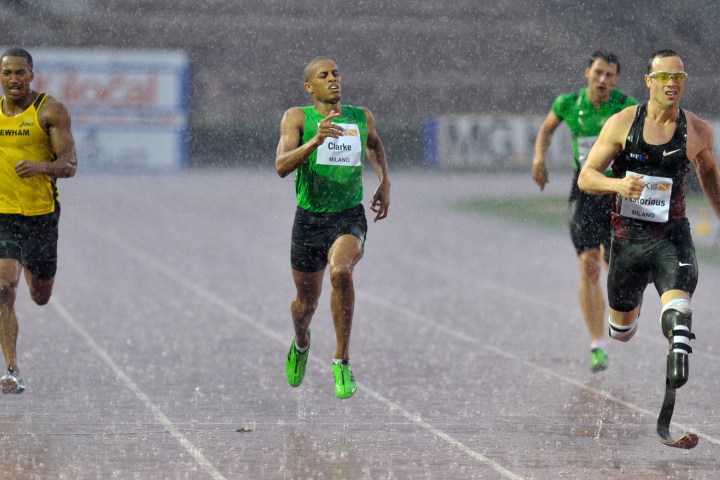The image captures a track and field competition in the midst of a torrential downpour, evident from the drenched competitors. Central to the scene is a runner named Clark, distinguished by his green tank top, black shorts, and green running shoes. His dampened bib confirms his name. He appears visibly strained, likely due to the challenging weather conditions. On his left, a runner in a yellow tank top and black shorts is also battling the elements. Foregrounded on the right, another competitor in a black tank top and shorts impressively runs with a prosthetic leg. Additionally, a man in a green shirt and black shorts, also wearing green shoes, can be seen in the background. The visibility is clear enough to discern these details, despite the rain blurring the overall scene. The runners are closely packed and display remarkable tenacity, with no spectators visible in the faded background of concrete steps and indistinct advertising.